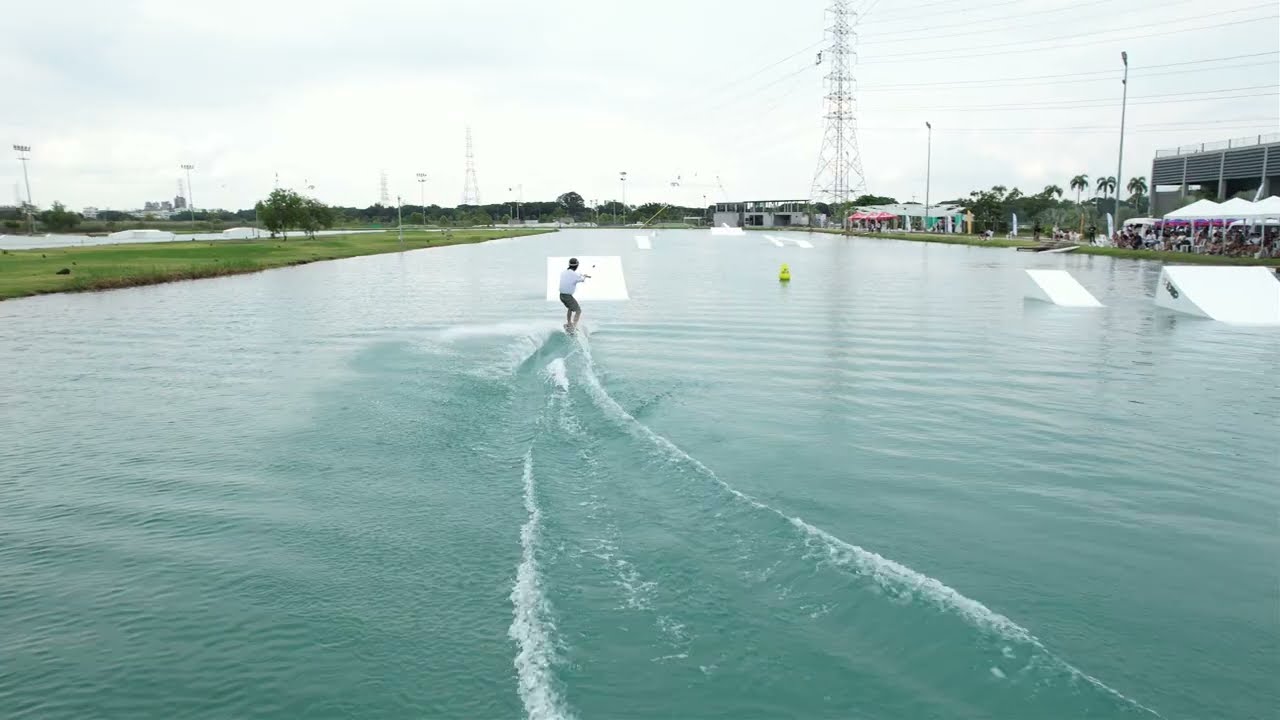This is a detailed color photograph taken outdoors at eye level, capturing a dynamic scene of a person engaging in water skiing. The central figure, slightly to the left of the frame, is a parasailor dressed in a white shirt and blue shorts. They are being pulled through a large, flat expanse of water by a kite, leaving a visible wake of ripples and waves behind them as they approach a prominent white ramp in the distance. Flanking the right side of the image, several more ramps can be seen, suggesting an area designed for water sports.

The setting appears to be a wide channel or canal, bordered by green grass and some ground. On the right coast, a crowd of spectators is gathered, sheltered under white pavilion-like tents, indicating that this might be an organized event or competition. Behind the spectators, there are low-lying gray buildings and tall palm trees. Extending into the background on the left are towering electrical structures, with several high-tension power lines stretching far into the distance, against a somewhat gloomy gray sky. The left side of the image also hints at a recreational area, marked by large sports lights over what might be a concrete field, adding to the overall ambiance of an active, bustling outdoor venue.